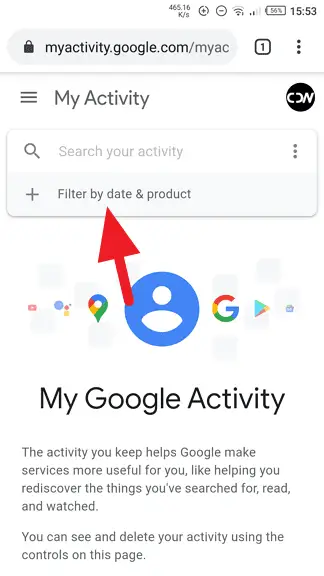In this screenshot, we observe the status bar at the top of a device's screen displaying several icons and indicators. The network signal strength is at 2 out of 4 bars, and there's a network speed meter depicting the current download or upload speeds. Additionally, the data saver icon, the do not disturb icon, and the WiFi signal icon showing 3 out of 4 bars are all visible. The device's time is 3:53 PM, and the battery level is at 56%. 

Below the status bar, a web page tab is open, displaying various elements related to Google activity. The title "My Activity" is prominently shown, with subsections titled "Search Activity," and a red arrow pointing towards "Filter by Date and Product." The page provides information stating, "My Google Activity: The activity you keep helps Google make services more useful for you, like helping you rediscover the things you've searched for, read, and watched. You can see and delete your activity using the controls on this page." This description offers guidance on how users can manage their digital footprint through the provided options.